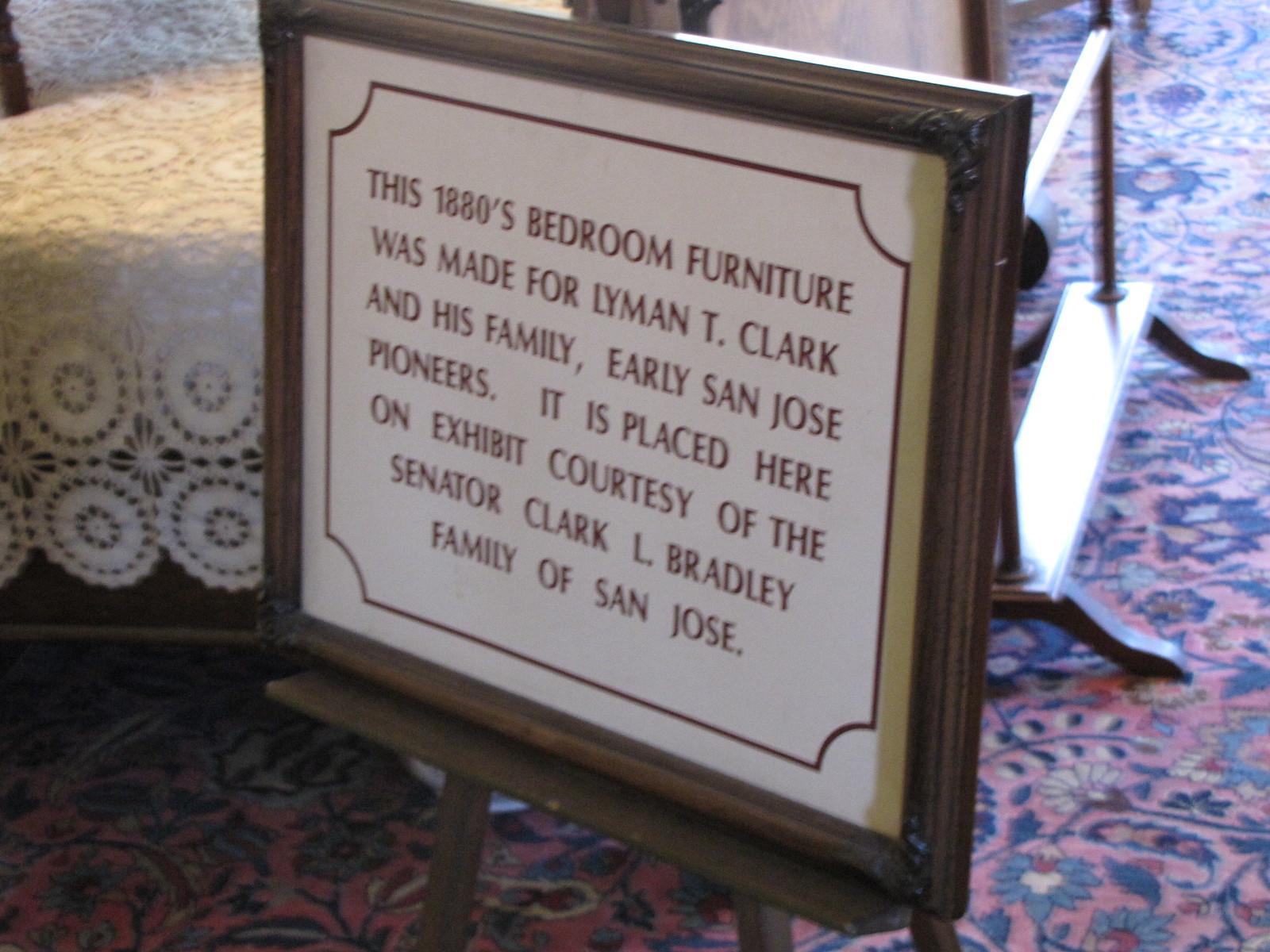This photograph, taken indoors, showcases a central wooden photo frame with rich dark brown staining and intricate scrollwork at the corners. The frame, which is resting on a matching wooden stand, elegantly encloses a piece of text against a light brown background. The inscription reads: "This 1880s bedroom furniture was made for Lyman T. Clark and his family, early San Jose pioneers. It is placed here on exhibit courtesy of the Senator Clark L. Bradley family of San Jose." The text is written in dark brown letters, framed by a thin, curved brown border that adds a touch of finesse.

The surroundings include a colorful carpet with floral motifs, which sets a historic ambiance. Behind the frame, other period-appropriate furnishings are visible, including a wooden bed adorned with a white doily-like bedspread. The setting appears to be part of a historical exhibit, capturing the essence of a late 19th-century bedroom, likely during the day. Various colors in the room include shades of brown, white, tan, pink, and hints of blue and yellow, all contributing to the image’s vintage aesthetic.